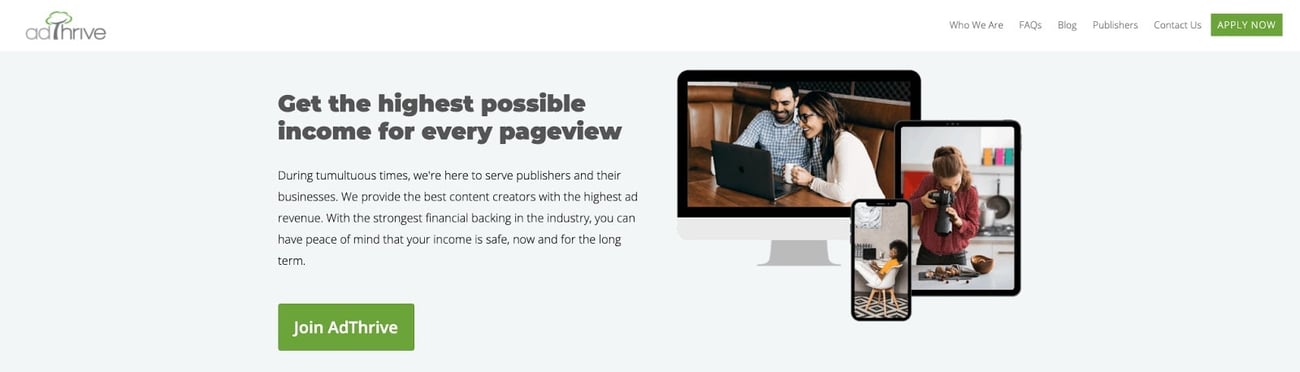This image features a website's homepage for Adthrive, showcased prominently with a logo in the top left corner where the "T" in "Adthrive" is creatively depicted as a tree. The navigation bar at the top is white and includes menu options such as "Who We Are," "FAQs," "Blog," "Publishers," and "Contact Us," along with a noticeable green "Apply Now" button. The main section of the page has a light blue background. On the right side of this central area, there are illustrations of a computer monitor, tablet, and cellphone, indicating the site's compatibility with various devices. On the left side, a section begins with the bold heading "Get the highest possible income for every page view," followed by a descriptive paragraph elaborating on the site's offerings.